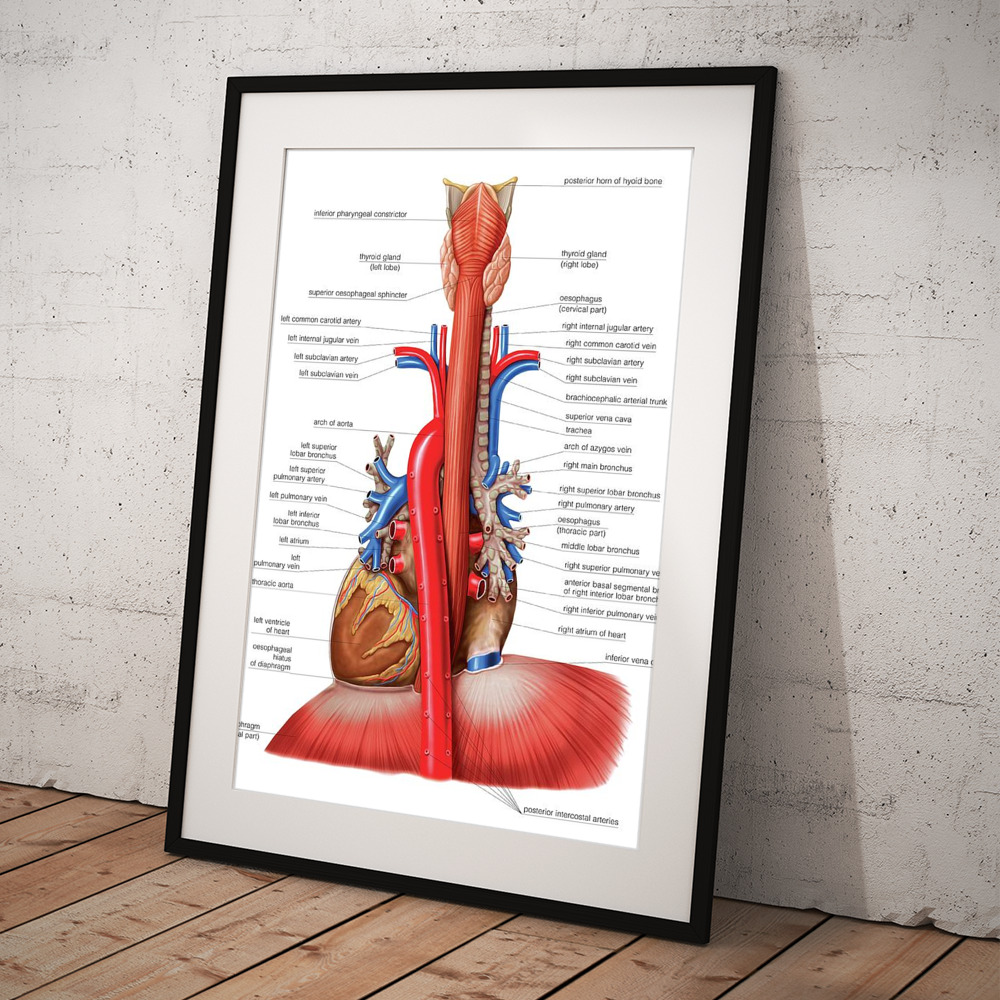The image depicts a large, detailed artist's rendition of the cardiopulmonary system, prominently featuring a variety of internal organs and vessels. The artwork, which includes labels for each part, is leaning against a white brick wall on a wooden floor, as if awaiting to be hung for educational purposes. The detailed illustration spans from the trachea through to the thoracic cavity, highlighting the heart and its numerous arteries and veins. Additionally, the artwork covers key structures such as the esophagus, thymus, lungs, and potentially other organs like the stomach, liver, or diaphragm. This medical representation is vividly colorful, meticulously labeled, and showcases the interconnectedness of the body's respiratory and cardiovascular systems.